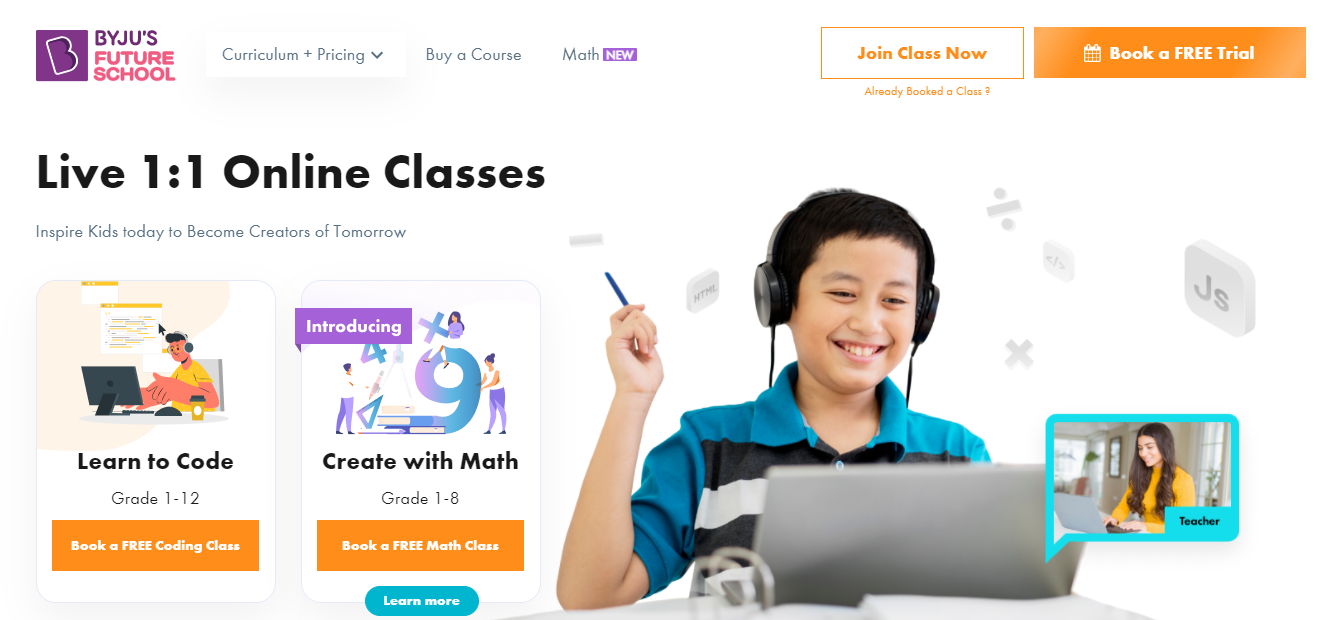This screenshot captures a webpage from BYJU'S Future School, set against a clean white background. At the very top-left corner, the company's name is prominently displayed with "BYJU'S" in bold purple text, followed by "FUTURE SCHOOL" in eye-catching pink, all in capital letters. To the left of the company name is a distinctive purple square logo with a white outline of the letter "B."

Directly below, the navigation menu features several items: "Curriculum + Pricing," "Buy a Course," "Math" (highlighted with a "New" label), and two rectangular buttons on the far right. The left button has a white background with the text "Join Class Now," while the right button features an orange background with "Book a Free Trial" in white text.

The main content of the website showcases a large, engaging photo on the right side. The image portrays a young Asian boy, around 10 years old, wearing over-the-ear headphones and a polo shirt with turquoise blue, black, and white horizontal stripes, seated before a silver-gray laptop.

On the left side of the screen, two colorful squares present the available courses. One square advertises "Learn to Code, Grade 1 to 12," while the adjacent square promotes "Create with Math, Grade 1 through 8." These vibrant elements contribute to an inviting and educational atmosphere on the webpage.